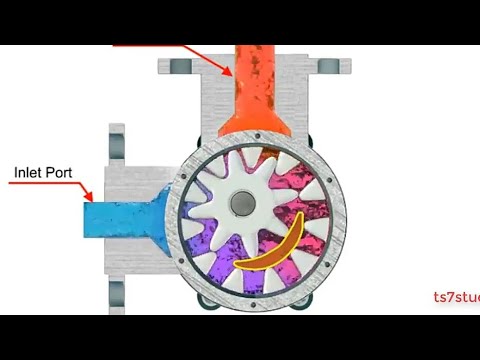The image is a low-quality frame from a video, digitally animated or synthesized, depicting a detailed illustration of a mechanical fluid pump. At the center of the image is a large gray circle with a set of interconnected cogs and gears. Notably, a central gear is connected to several cogs located in the top right portion of the circle. Inside this circle, a purple and pink liquid can be seen, suggesting the fluid being pumped. Above the circle, there is a metal piece showing a red liquid flowing into the space, indicated by a red arrow pointing to this inlet port, which has "inlet port" labeled in black writing. A similar metal piece on the left side shows a blue liquid flowing into another inlet port. The bottom right corner contains partially visible red lettering "TS7STU," which extends off the screen. The background is plain white, and both the top and bottom of the image are bounded by black bars, giving it a frame-like appearance.